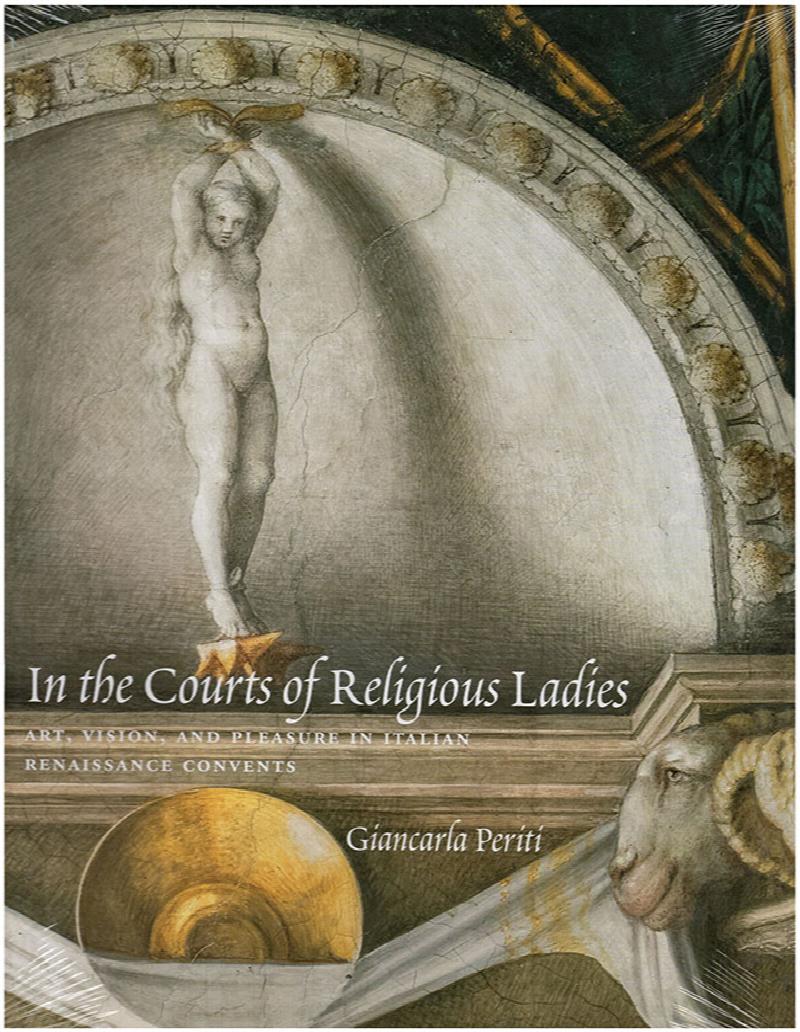This color image appears to be the cover of a book or a poster for an art exhibition, featuring a detailed painting evocative of Italian Renaissance art. Central to the composition is a painting of a cherub, apparently female, with long hair and her arms tied above her head at the wrists with a yellow ribbon. She stands within a white circle, under a white arch adorned with small, shell-shaped medallions. The cherub appears to be standing on a pediment, atop what seems like intricate, aged stonework, evidenced by visible cracks. Beneath this scene, in white text, is the title "In the Courts of Religious Ladies: Art, Vision and Pleasure in Italian Renaissance Convents," with the author's name, Giancarlo Peridi, also in white text on the bottom right. The artwork also includes a gold semicircle resembling a halo and features carvings, including a ram, adding to the ornate and historical nature of the design.